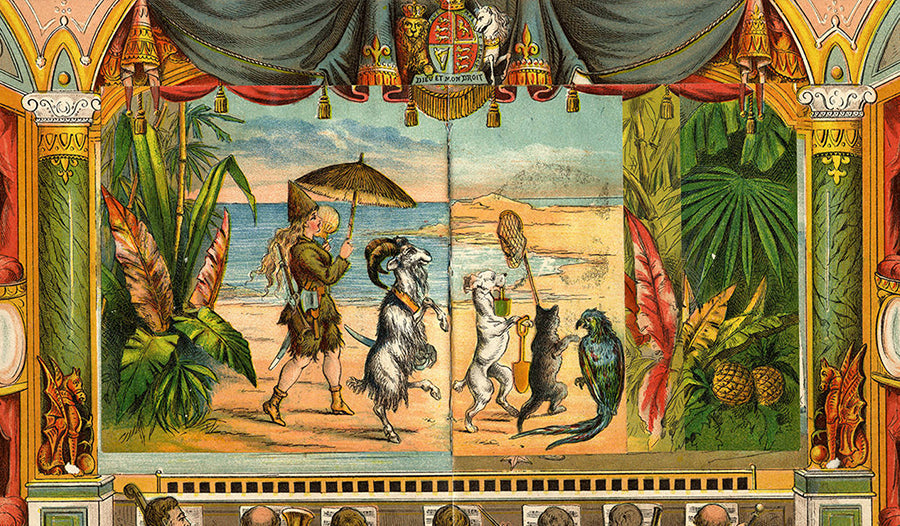The artwork depicts a whimsical scene reminiscent of a child's storybook, featuring a blend of fantastical and possibly British colonial elements. Central to the horizontal composition is a shoreline setting where an array of anthropomorphic animals and a human figure walk in a parade-like manner. The backdrop suggests a theatrical stage with ornate details. 

On this beach, amid tan sands, a white goat with arcing horns and a sword at its waist leads the procession, followed by a white dog carrying a green basket in its mouth and a yellow shovel in one paw. A dark gray cat, moving towards the right but with its back to the viewer, holds a net on a pole. Lastly, a parrot perches on the far right, standing still. Following the animals is a human figure, possibly a woman or adolescent, dressed in an olive green, triangular-shaped hat, tattered shorts, and yellow boots. The figure carries a fan made of feathers, a straw umbrella, and is equipped with a hatchet, a rifle, and a sword.

Above this scene, the sky is blue with tinges of gray and pink, suggesting a serene sunrise or sunset. Calm blue water stretches into the horizon, met by a faint hill in the distance. On either side of the stage, tropical foliage frames the scene, including green bamboo, triangular leaves, and red fronds, with two pineapples nestled among the greenery on the right.

The theatrical elements include an elaborate stage frame with green marble columns topped with detailed white stone caps and gold accents. Gold and red curtains drape from above, alongside black and ornate fabric banners adorned with gold tassels and red and gold arcs. Centered above the scene is a royal coat of arms featuring a gold lion and a white unicorn beside a divided red shield. Below the stage, musicians—presumably Caucasian men—are depicted playing instruments, amidst scattered music sheets. The boundaries of the artwork include intricate arches and shelves, presenting a semblance of a royal and exotic tableau.